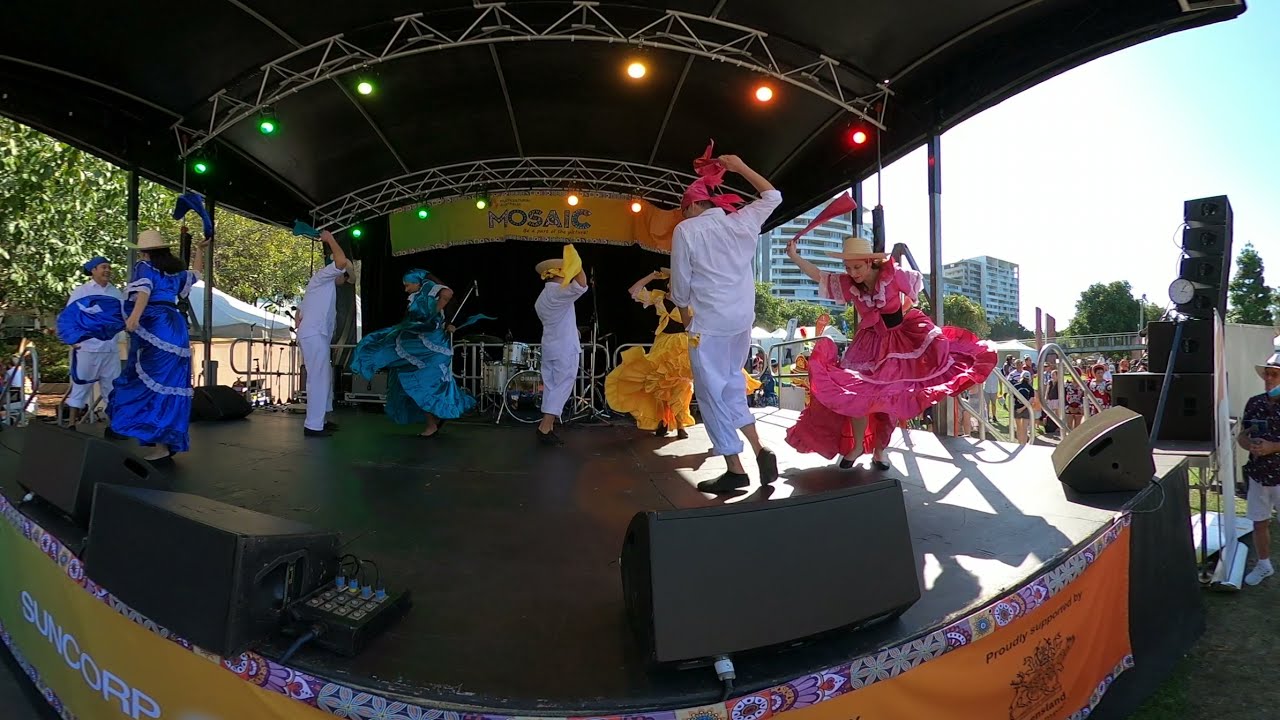The image captures an outdoor performance on a portable, elevated stage with a black surface, framed by an orange banner that reads “SunCorp” on the left and “proudly sponsored by” on the right, accompanied by an emblem. A fisheye lens or 360-degree effect distorts the scene, revealing an overhead metal structure supporting stage lights. Men in traditional Mexican peasant attire—white pants and shirts with matching colored bandanas—dance energetically alongside women in vividly colored, flowing ruffled dresses, ranging in hues of neon blue, pink, yellow, and white, and wearing straw hats. The vibrant scene is bathed in bright sunlight, casting distinct shadows. A yellow sign reading “Mosaic” hangs on the back wall, with a drum set visible below it, though the drummer is absent. In the background, there are trees, a pop-up tent on the left, and a crowd of other people on the right, with multi-story buildings and a partly blue sky visible in the distance.